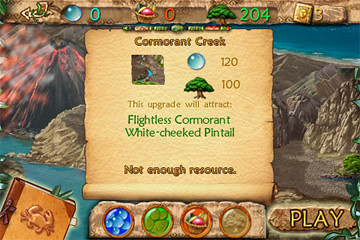In the image, we observe a video game interface. The top of the screen is adorned with brown rock formations and several icons. From left to right, the icons include a blue circle followed by the number zero, a red planet encircled with gold coupled with a red zero, and a green bush with the number 204 in green text beside it. Further to the right, there are some textual elements that are not fully legible. Moving to the background of the screen, the upper right corner features water, while substantial gray rocks occupy a significant portion of the scene. 

There are visual effects that suggest shots being fired, with red and gray flames and smoke emanating from the activity. At the bottom of the screen, there is a depiction of a little crab situated in front of what appears to be a book. Next to this, there are four colored circles — blue, green, red, and brown — and a "Play" button is prominently displayed.

Centrally located on the screen is a beige-colored square labeled "Camorant Creek," which includes resource indicators: 120 beside the blue circle and 100 next to the green tree. Notably, the words "flightless Camorant" and "white-cheeked pintail" are displayed, alongside the message "not enough resource."